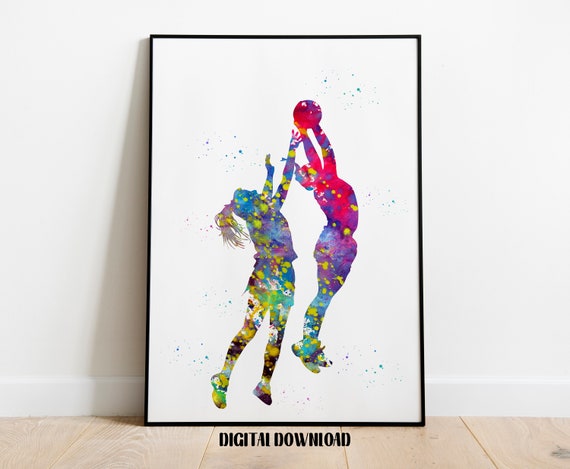This image features a vibrant painting of two colorful, futuristic characters engaged in a dynamic game of basketball. The character on the right, leaping into the air to dunk the purple and red basketball, is depicted in a spectrum of blue, yellow, green, red, and purple hues. Their movement is fluid and full of energy, showcasing an artistic pose that emphasizes their athleticism. On the left, a character with a ponytail reaches up, attempting to intercept the dunk. Similarly adorned in a palette of green, yellow, blue, and red, both characters are distinct yet harmoniously colorful. The vivid brush strokes and paint splatters enhance the sense of motion and intensity of the game. The background is a stark white sprinkled with blue specks, creating a contrast that makes the characters pop. Framed in black, the painting is captioned with the black text "digital download" at the bottom. The scene is set against a room with white walls and beige flooring, adding to the painting's prominence and focus within the image.